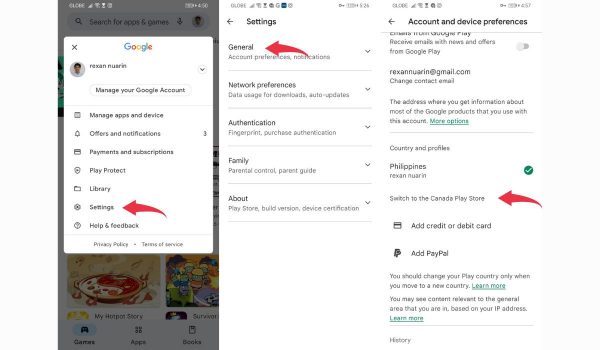The image comprises a series of three sequential screenshots from the Google Play Store, displayed side by side, each containing detailed interface elements primarily related to account management and settings.

**Screenshot 1:**  
The first screenshot shows the main interface of the Google Play Store, with a grayed-out background indicating the Play Store interface. It includes a search box with a magnifying glass icon, a microphone icon, and an indistinct profile picture icon at the top. The top of this screenshot also vaguely displays the current time and blurry game-related imagery along with tabs for 'Games,' 'Apps,' and 'Books.' Superimposed on this screen is a pop-up window featuring the Google logo in blue, red, yellow, and green colors, with an 'X' at the top corner for closing the pop-up. It displays the user's username and profile picture. Below that, sections such as "Manage your Google Account," "Manage apps and device" with a paper icon, "Offers and notifications" with a bell icon showing three notifications, "Payments and subscriptions" with a credit card icon, "Play Protect" with a shield icon, "Library" with a manila folder icon, "Settings" with a cogwheel icon highlighted by a red arrow, and "Help and feedback" with a circle icon. Additionally, the footer includes "Privacy Policy" and "Terms of Use."

**Screenshot 2:**  
The second screenshot delves into the settings menu of the Play Store, displayed over a white background with black font. It features a back arrow at the top, indicating navigation to the previous screen. The title "Settings" is clearly visible. Below it, various sections such as "General" highlighted by a red arrow, "Account preferences and notifications," each accompanied by a pull-down arrow. Other sections include "Network preferences" detailing data usage for downloads and auto-updates, "Authentication" listing fingerprint purchase authentication options, "Family" indicating parental controls and a parent guide, and "About" which includes Play Store build version and device certification. 

**Screenshot 3:**  
The third screenshot focuses on "Account and device preferences," also displayed on a white background with black text. It includes the user’s Gmail address beside a gray profile circle and a brief description about receiving information related to Google products associated with the account. Following this, there is a section labeled "Country and profiles." It shows the current country, Philippines, marked with a green check mark, and a red arrow pointing to an option for switching to the Canada Play Store. Payment options like "Add credit or debit card" with a credit card icon and "Add PayPal" with a PayPal 'P' icon are visible. At the bottom, information in gray text advises users to change their Play country only when they relocate to a new country, accompanied by a teal box link labeled "Learn more." It also mentions user location determination based on IP address, followed by a final "Learn more" box and a "History" label in gray at the bottom.

These screenshots provide a comprehensive visual guide to various settings and account management options available on the Google Play Store.